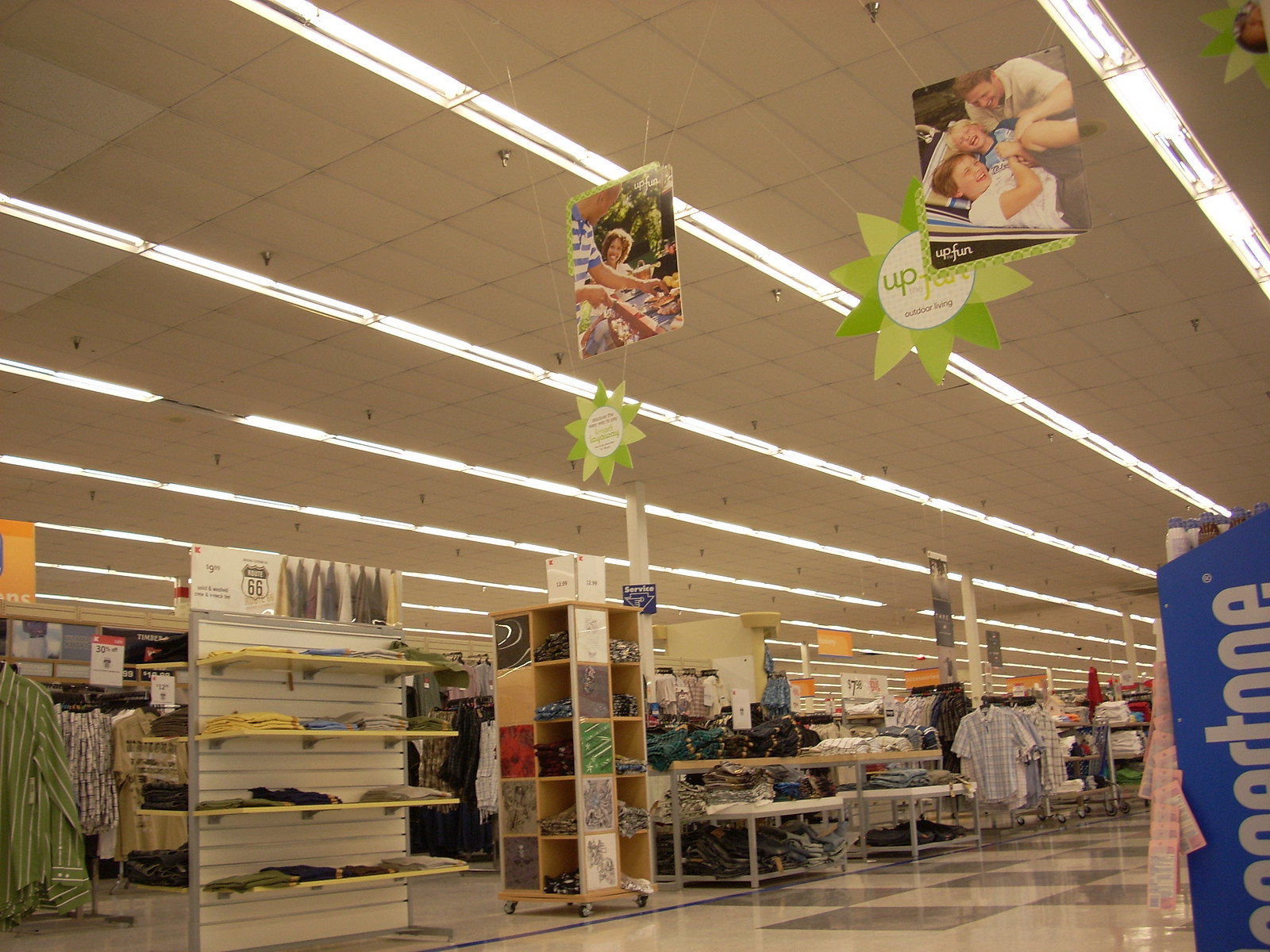This image depicts a section of a department store dedicated to clothing. The store features neatly organized shelves and desks with folded garments, alongside racks displaying a diverse array of colorful clothing. The ceiling is white, adorned with evenly spaced lights illuminating the space. The store's flooring varies, with a checkered linoleum pattern leading into a plain gray area beneath the clothing displays. Suspended from the ceiling are vibrant advertisements showcasing families engaged in various joyful activities, highlighting the clothing available in the store.